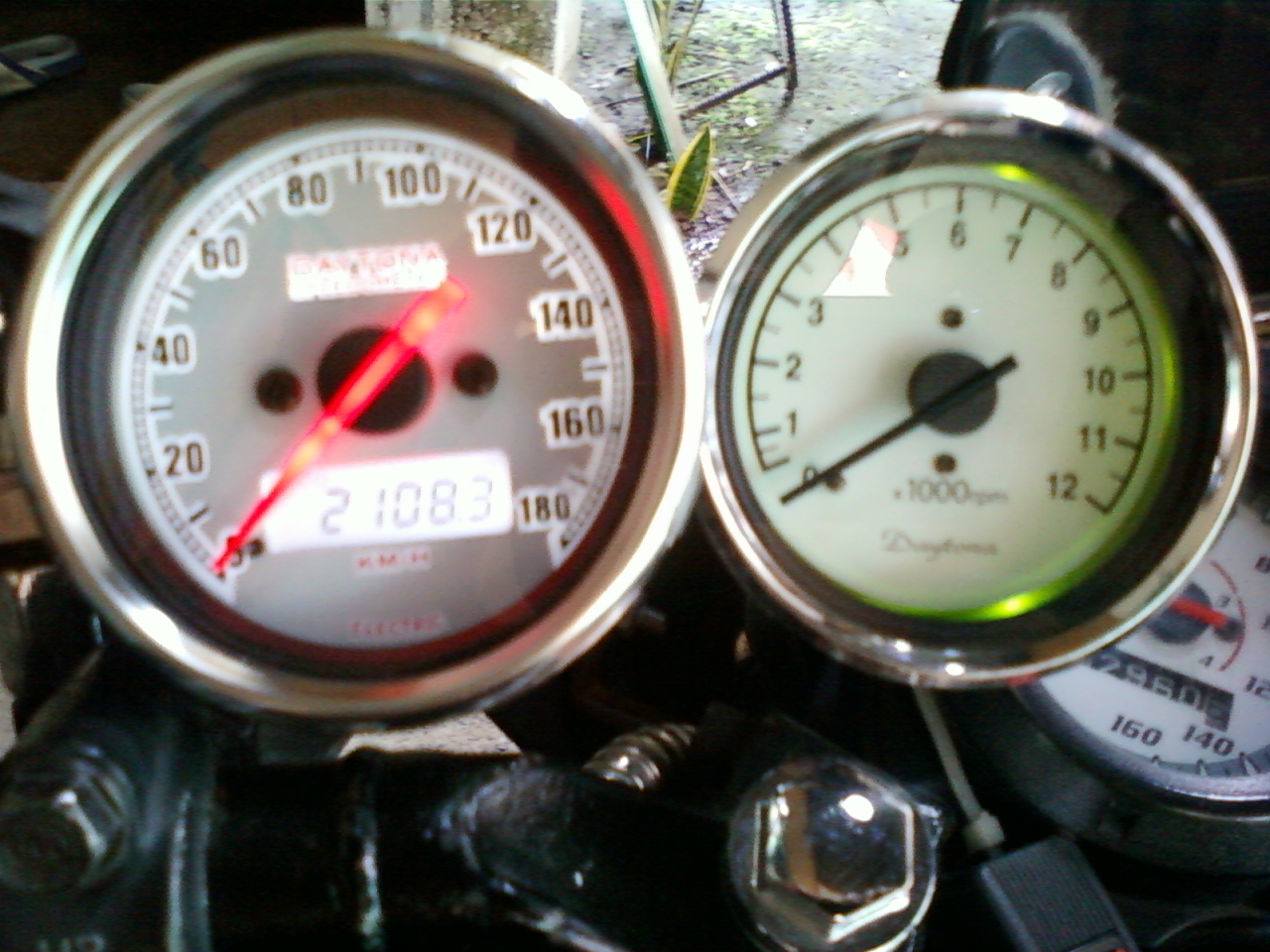This landscape-oriented photograph captures a collection of detached speedometers situated in what appears to be a mechanic’s garage. Two prominent speedometers dominate the scene, positioning themselves centrally. The left speedometer, encased in a steel border with a gray interior, is distinctly illuminated, and its red dial hand stands out sharply. Adjacent to it, the right speedometer also features a steel border, glowing with a green hue, and is accented by a black dial hand against its white background. In the bottom left corner, partially obscured by the two larger speedometers, a smaller third speedometer is visible. The top of the frame offers a glimpse of the outdoors; the bright daylight filtering through reveals a yard outside the garage. The overall image has a slightly blurred quality, adding an atmospheric touch to the setting, where the speedometers rest atop various black objects and tools, further signaling the industrious environment of a garage workspace.